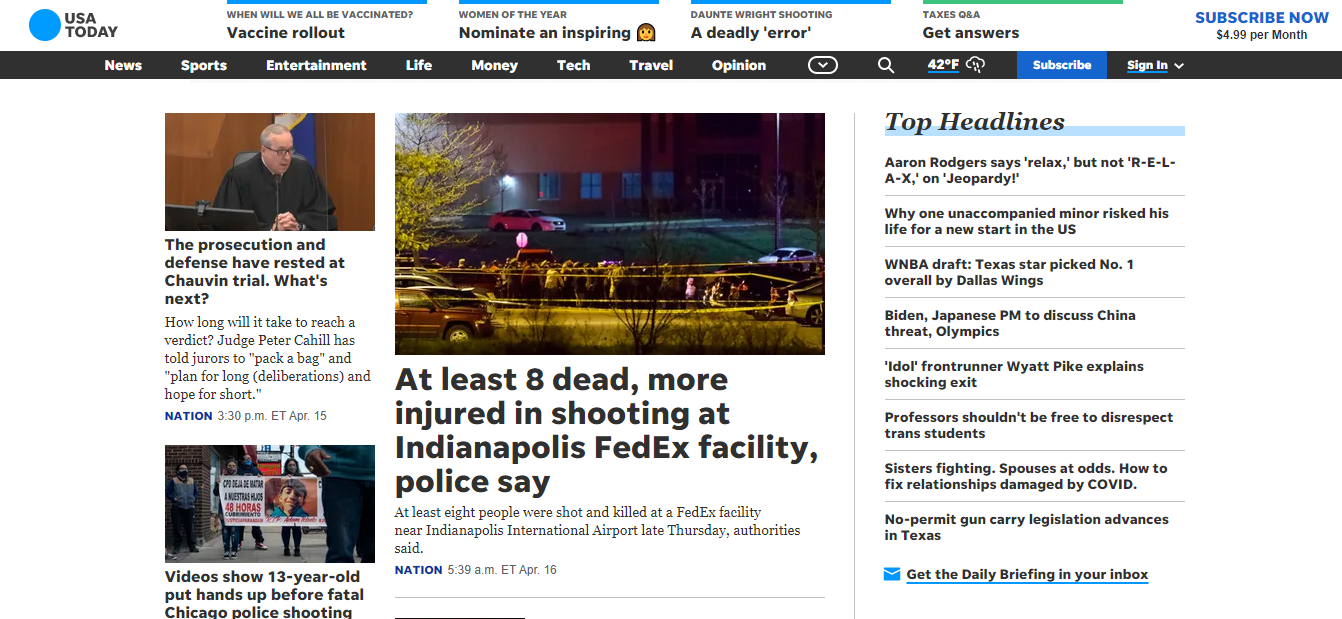The screenshot depicts a webpage from the USA Today website as viewed on a computer. The main focus of the page includes an option to subscribe for $4.99 per month. 

At the top, four highlighted news snippets are displayed horizontally:
1. "When Will We All Be Vaccinated?" with the subtitle "Vaccine Rollout."
2. "Woman of the Year," encouraging readers to "Nominate an Inspiring Woman" accompanied by an emoji.
3. "Daunte Wright Shooting," described as "A Deadly Error" in quotations.
4. "Texas Q&A," distinguished by a green line at the top as opposed to the blue lines on the other three, with the text "Get Answers" underneath.

Beneath these snippets, there is a black horizontal menu bar featuring various categories such as News, Sports, Entertainment, Life, Money, Tech, Travel, Opinion, and an arrow indicating more options. The current weather is displayed, showing 42°F and rainy conditions. Additionally, the page provides options to "Subscribe" or "Sign In."

The top headline is prominently featured, reading "At Least Eight Dead, More Injured in Shooting at Indianapolis FedEx Facility, Police Say." This headline suggests the events are current, around April 15-16. The overall theme of the news stories revolves primarily around shootings and related incidents.